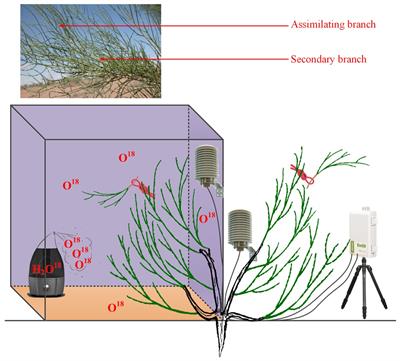The image presents a scientific diagram interspersed with a photograph and detailed annotations. In the upper left-hand corner, a photograph showcases a sand dune with a long green plant. The plant has slender stems, labeled with red arrows indicating as "Assimilating branch" and "Secondary branch." Beneath this photograph is a large, detailed diagram. This diagram features a cube with purple walls and a tan base, displaying a replication of the plant from the photograph, situated centrally. To the left within the cube, there's a black apparatus marked with "O18," accompanied by small, unreadable numbers. Additionally, two large white cylindrical objects are drawn surrounding the plant. On the far right of the diagram stands a black tripod supporting a white box, seemingly monitoring the plant’s interaction with the cube. This intricate depiction suggests a scientific setup, possibly from a textbook, with elements of real-life application and diagrammatic representation.